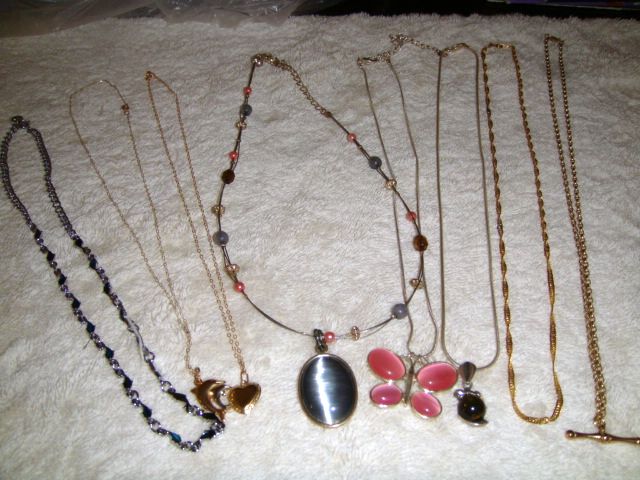The image captures a slightly out-of-focus, color snapshot of a soft, white shaggy throw rug, likely placed in a bathroom or next to a bed. Despite the glaring light at the bottom, the primary focus is on a collection of eight necklaces meticulously spread out across the rug. The upper left corner of the image shows a clear plastic bag crumpled on the rug. The necklaces, ranging in length from approximately 16 to 24 inches, exhibit a variety of designs and materials, suggesting they may date back to the early to mid-2000s.

From left to right, the detailed descriptions of the necklaces are as follows:
1. A silver-tone chain adorned with faux abalone dolphins.
2. A gold-tone chain featuring either a fish or a dolphin pendant.
3. Another gold-tone chain with a heart-shaped pendant.
4. A cable-style chain with an adjustable section near the neck, embellished with different colored glass beads and a prominent oval pendant.
5. A thin silver-tone chain with a butterfly pendant made of four pink resin stones.
6. Another thin chain with a spherical black bead mounted intricately.
7. A twisted gold-tone chain with a hammered-flat appearance.
8. A ball chain reminiscent of a pull chain, ending with a pendant resembling a double-sided bowling pin.

The collection appears quite dated and might suggest an informal display, perhaps hinting they are for sale or simply showcased. The necklaces vary in their level of intricacy and adornment, ranging from simple metallic designs to those featuring colorful beads and distinctive pendants.